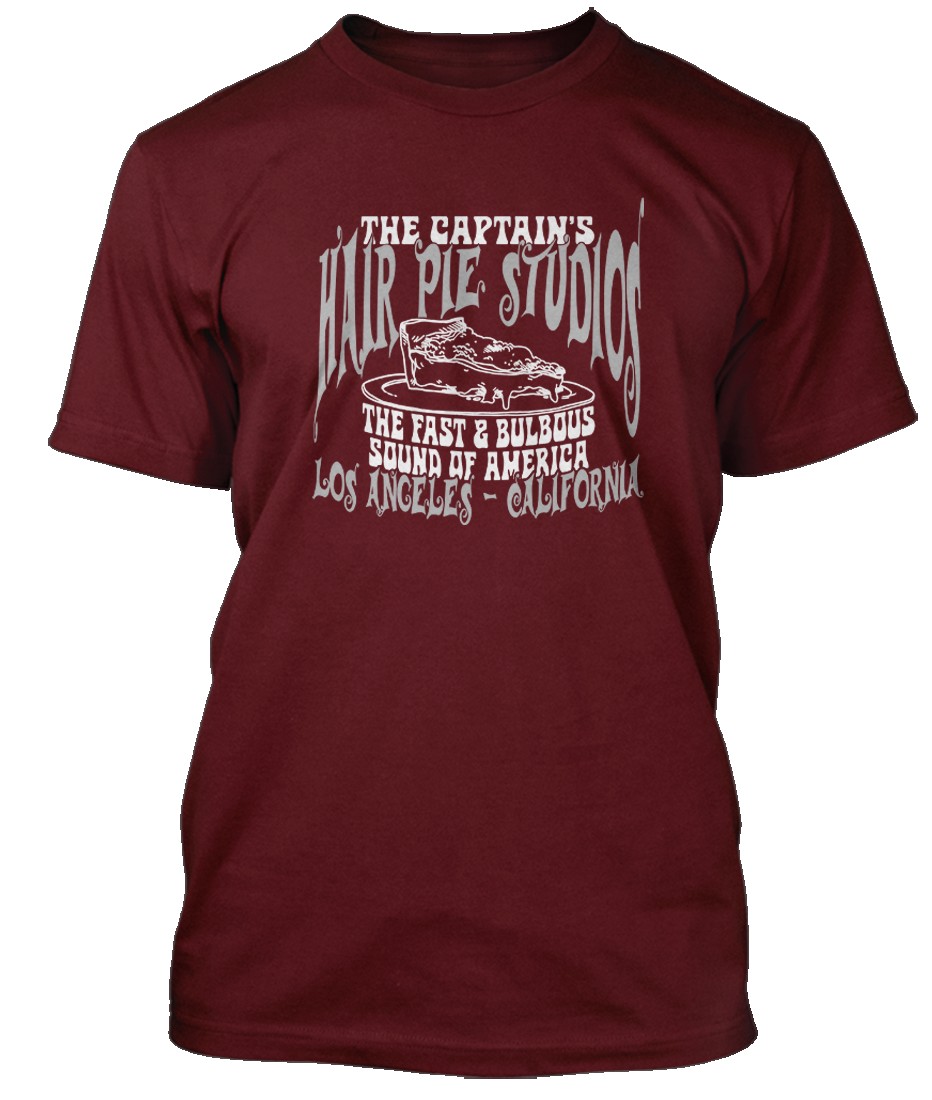This is a detailed image of "The Captains" t-shirt, featured as it would appear in a clothing catalogue from a brand website. The shirt is a maroon, dark red, purplish color and designed for males, as suggested by its fitted chest area and broad shoulders. It is a typical short-sleeved t-shirt with a regular rounded neckline.

The front of the shirt showcases an elaborate, all-caps, curly font in white and gray. At the top, it reads "The Captain's," followed by a larger, curved inscription of "Hair Pie Studios." Centrally positioned below the text is a white depiction of a slice of pie on a plate. Beneath this image, in white lettering, it says "The Fast and Bulbulous Sound of America." 

Further down, in a similar swirly font but gray in color, it reads "Los Angeles, California." The text and imagery are strategically placed on the chest area, fitting neatly within the bounds of the t-shirt's short sleeves. The background of the image is entirely white, emphasizing the vivid maroon color and intricate details of the shirt.